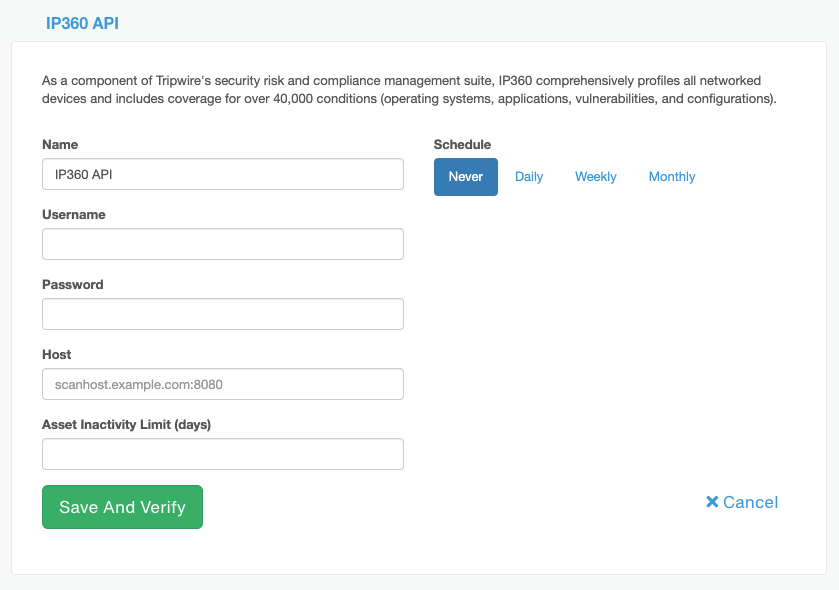This image is a screenshot of the IP360 API section of a website, which is a component of Tripwire's security risk and compliance management platform. 

**Header and Introductory Text:**
- At the very top left corner, bold blue text prominently displays "IP360 API". 
- Directly below this, there is a smaller font paragraph explaining the purpose of IP360. It states: "As a component of Tripwire security risk and compliance management site, IP360 comprehensively profiles all network devices and includes coverage for over 40,000 conditions (operating systems, applications, vulnerabilities, and configurations)."

**Form Fields:**
- Following the introductory text, the page presents a series of input fields arranged vertically for user interaction:
  1. **Name:** A text box labeled "Name" with "IP360 API" pre-filled with black text.
  2. **Username:** An empty text box labeled "Username".
  3. **Password:** An empty text box labeled "Password".
  4. **Host:** An empty text box labeled "Host".
  5. **Asset Inactivity Limit (days):** An empty text box labeled "Asset Inactivity Limit (days)".

**Action Buttons:**
- At the bottom left-hand corner, there is a green button labeled "Save and Verify".
- To the right of the green button, there is a blue button labeled "Cancel (X)".